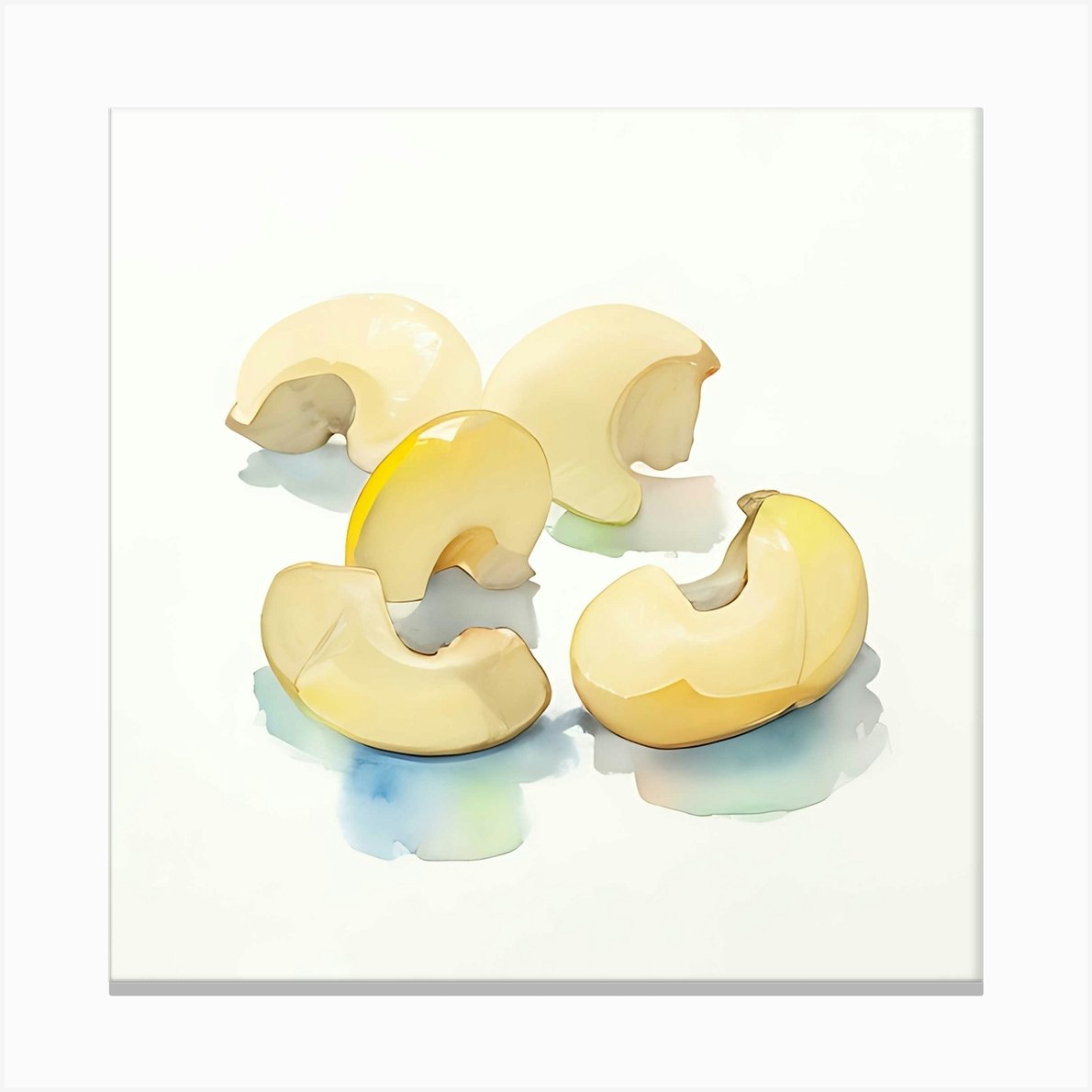This image features a watercolor painting nestled within a very light gray frame. The outer frame measures approximately 6 inches high by 6 inches wide, with a thin, light gray border surrounding a slightly inset light gray background. Within this background, positioned centrally, is another smaller, square image about 4 inches on each side. This inner image has a slightly thicker light gray border, predominantly along the right side and bottom edge, framing a white background.

The painting itself depicts five irregularly shaped objects that evoke the appearance of either broken eggshells, cashew nuts, or beans. Each shape features a yellow-tinted outer rim, transitioning to an off-white with cream undertones towards the center. The subject has a soft, delicate quality, likely due to initial pencil sketches underneath the watercolor. Each object is paired with a subtle shadow effect, rendered in watercolor shades of green, blue, pink, and red, giving the impression that the objects are slightly elevated from the background. These shaded hues create a gentle, almost ethereal atmosphere, enhancing the beige and yellow accents of the objects themselves.